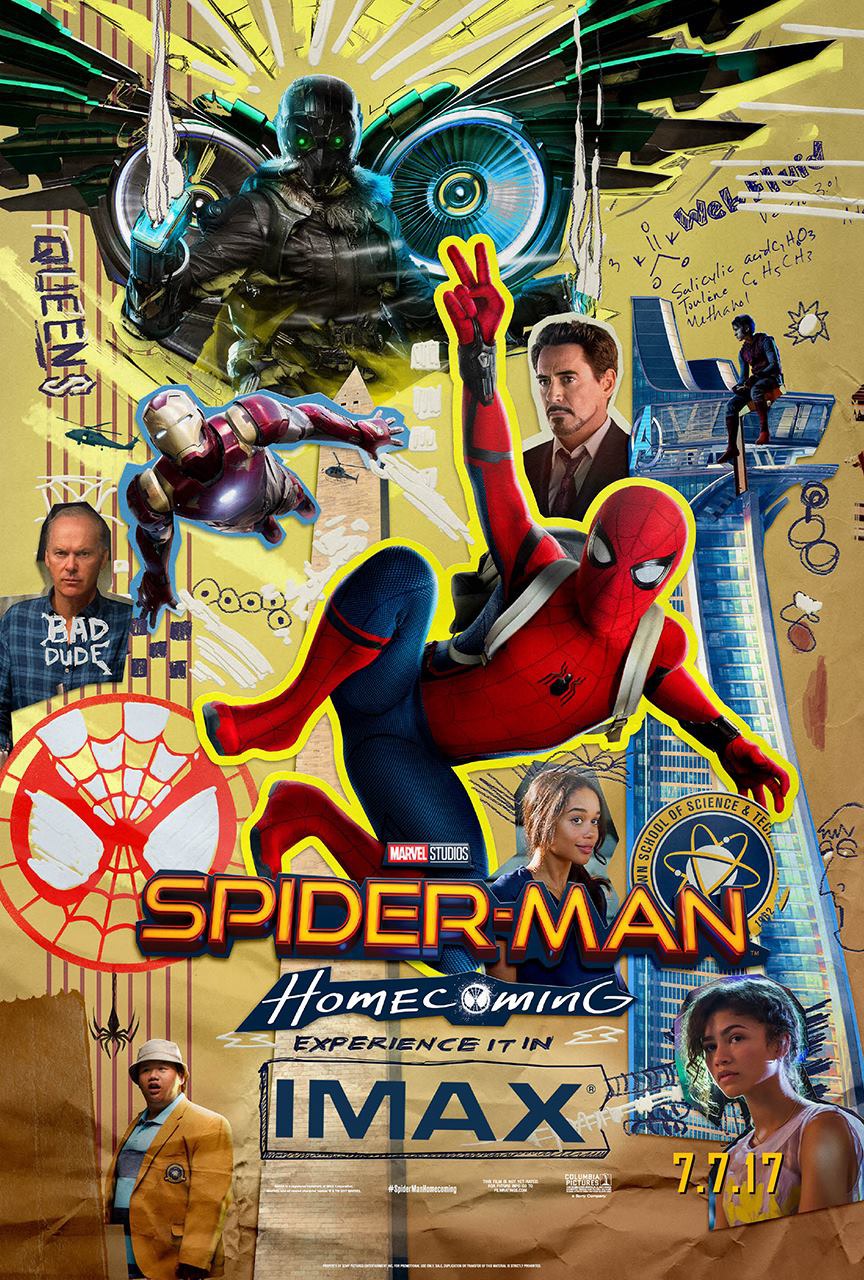This vibrant, comic book-style movie poster for *Spider-Man: Homecoming* features Spider-Man front and center, dynamically posed as if soaring through the air with a backpack on and flashing a peace sign with his right hand. His iconic red suit, blue pants, red boots, black webbing, and distinctive white eyes are detailed prominently. Hovering behind him is Iron Man, depicted mid-flight. The poster also showcases Robert Downey Jr. twice: once as Iron Man and once in his civilian attire. 

At the top left, we see a menacing figure, possibly the Vulture, clad in black armor with large black wings and green eyes, wielding a black and silver sword. Below Spider-Man, the poster includes images of two female actresses, potentially Michelle Rodriguez and Zendaya, and an Asian male actor wearing a hat. The entire design features a colorful, collage-like array of characters and cutouts, reminiscent of a sketchbook aesthetic.

The bottom of the poster is marked with prominent text: “Marvel Studios Spider-Man: Homecoming. Experience it in IMAX 7.7.17,” indicating the movie's release date and format.